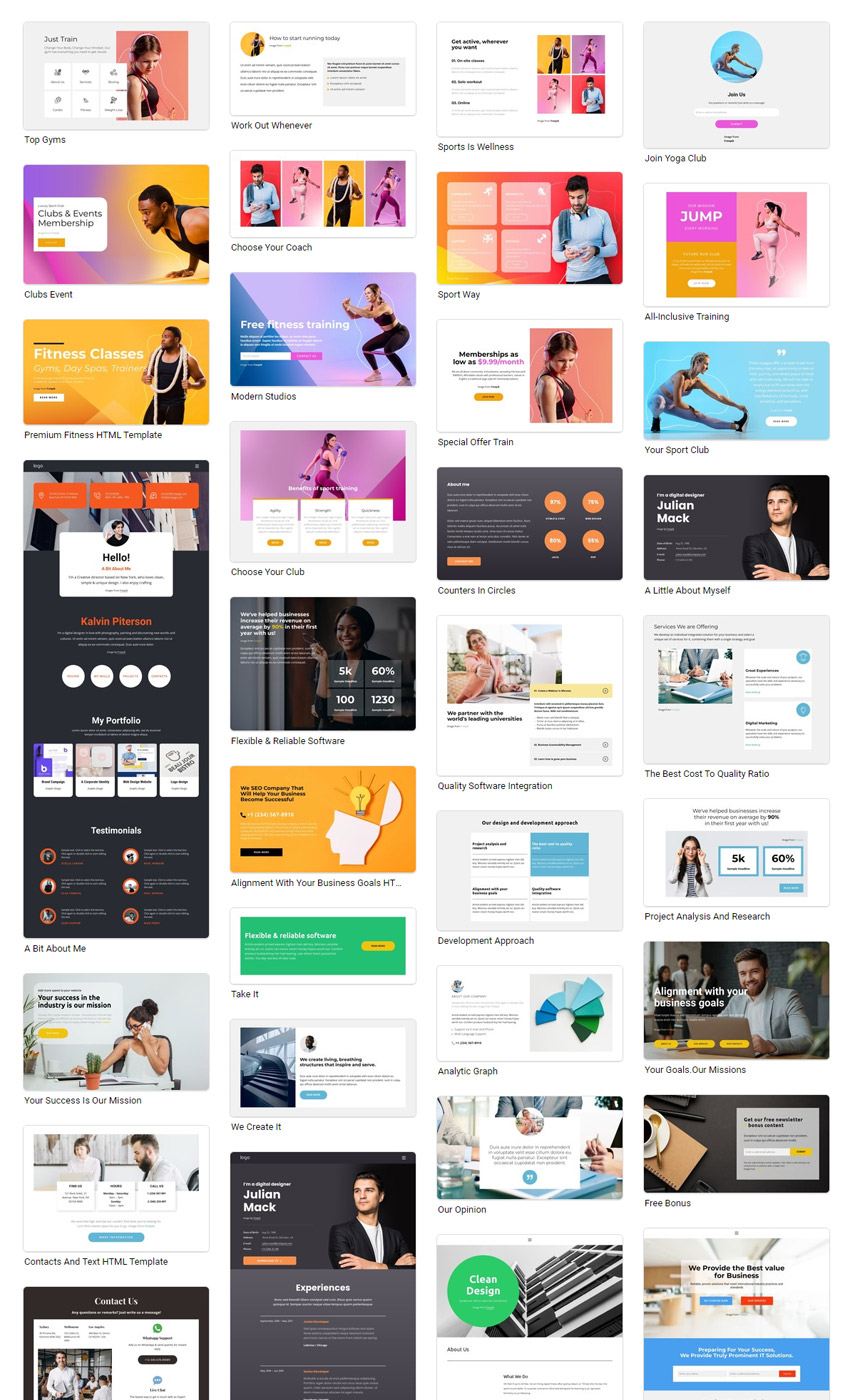This image selection, organized left to right and top to bottom, is a comprehensive showcase of diverse fitness and wellness themes, featuring an array of vibrant and engaging visuals:

1. **Top Gyms**: A woman wearing earphones, likely preparing for an intense workout session.
2. **Workout Whenever**: Highlighting the flexibility of gym schedules.
3. **Sports as Wellness**: A collage of photographs capturing various individuals engaged in different workout routines, emphasizing the importance of physical activity for overall wellness.
4. **Join Yoga Club**: A serene image of someone stretching, inviting viewers to join a yoga community.
5. **Clubs Event**: A powerful shot of a dark-skinned man doing pushups, exemplifying strength and endurance.
6. **Choose Your Coach**: Multiple images of people working out, suggesting personalized coaching options.
7. **Sport Way**: A light-skinned man absorbed in his cellphone, possibly reviewing his fitness progress or workout plan.
8. **All-Inclusive Training**: A dynamic photo of a woman mid-jump, promoting the inclusivity of the training programs.
9. **Fitness Classes**: A dark-skinned man with a towel draped around his neck, looking contemplatively to the left, symbolizing the dedication and focus in fitness classes.
10. **Modern Studios**: A woman performing squats in a modern fitness studio, showcasing the facility’s state-of-the-art equipment.
11. **Special Offer Train**: A fair-skinned woman with headphones looking downward, possibly during a moment of rest or contemplation.
12. **Your Sport Club**: Another fair-skinned woman stretching, reflecting the inclusive and community-driven nature of the sport club.
13. **A Bit About Me**: Personalized introductions, potentially for fitness trainers or coaches.
14. **Choose Your Club**: A fair-skinned woman lifting weights, highlighting strength training options.
15. **A Little About Myself**: A fair-skinned young man with his arms crossed against his chest, looking to the left, signifying confidence and readiness.
16. **Flexible and Reliable Software**: Emphasizing the adaptability and dependability of the fitness software.
17. **Quality Software Integration**: Assurance of high-quality software solutions for fitness club management.
18. **The Best Cost to Quality Ratio. Alignment with Your Business Goals**: Depicted with a line drawing of a white head with a light bulb emerging from it, symbolizing innovative and cost-effective solutions.
19. **Project Analysis and Research**: Focuses on the analytical aspect of business planning.
20. **Take It. Your Success is Our Mission. We Create It.**: Accompanied by an analytic graph, underlining a commitment to client success.
21. **Your Goal is Our Mission**: Featuring a light-skinned man working on a laptop, representing the tailored approach to achieving fitness goals.
22. **Contacts and Text HTML Template**: Possibly showcasing contact information or features of an HTML template.
23. **Our Opinion**: Sharing expert insights or reviews.
24. **Free Bonus**: Offering additional value or incentives.
25. **Additional Options**: Other options are present but cut off at the bottom edge of the screen.

This detailed description captures the essence and diversity of the images, effectively conveying the multifaceted approach to fitness, wellness, and related technological integrations.